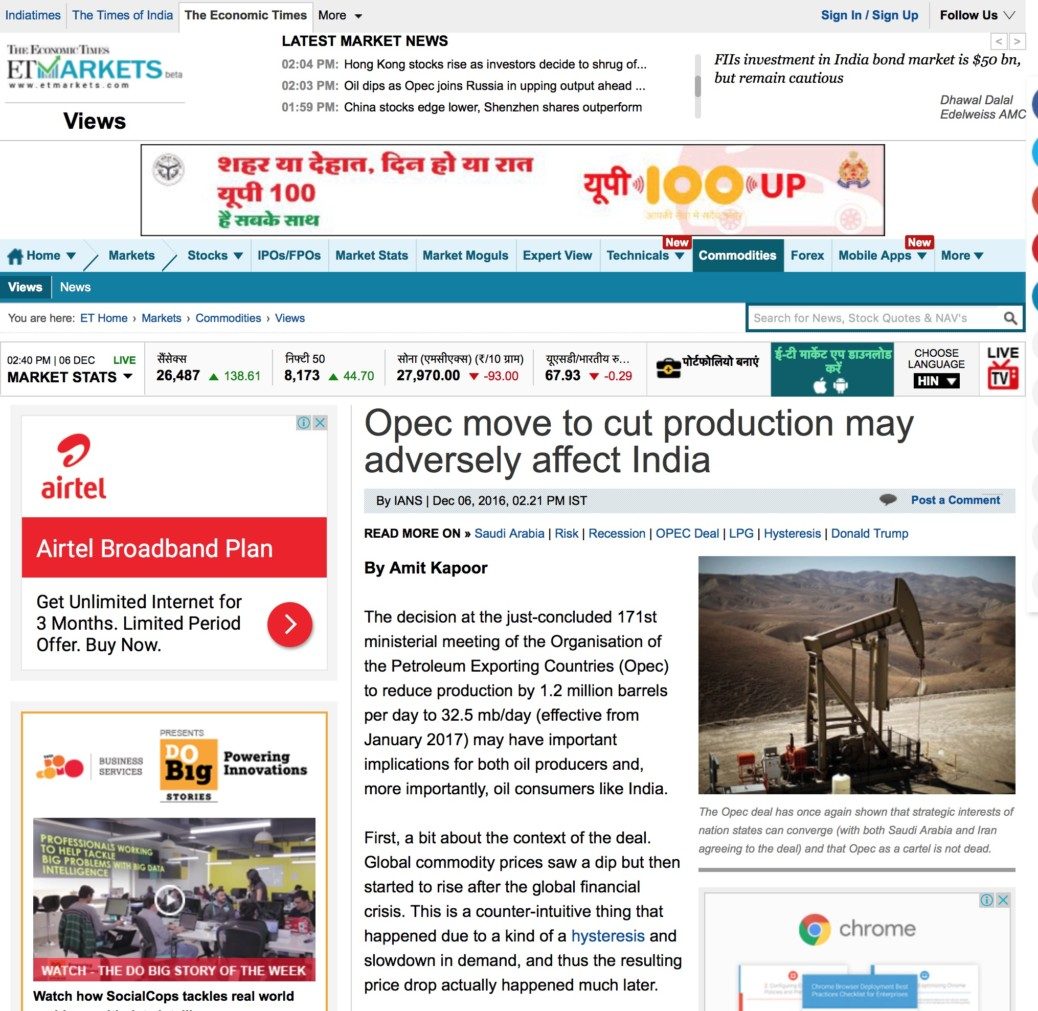The webpage being described is part of ET Markets, a sub-section of the Economic Times website. The header prominently displays "Economic Times" (ET) with options to navigate to the Times of India and India Times websites, alongside a "More" button. The ET Markets section is highlighted, indicating it is in beta phase and not fully open to the public. 

The ET logo features 'ET' in bold, while the 'Markets' section has a unique 'M' that resembles a fluctuating stock market graph in turquoise color. The domain "etmarkets.com" is displayed underneath.

Below this, there’s a bold heading "Views," and to the right, under the Economic Times tab, another bold heading reads "Latest Market News." Listings of current news items follow, each showing a timestamp:
- 2:04 PM: "Hong Kong stocks rise as investors decide to shrug off."
- 2:03 PM: "Oil dips as OPEC joins Russia upping the output."
- 1:59 PM: "China stocks edge lower."

To the far right, there's a headline "F2's Investment in Indiana Bond," and the top right corner features options to "Sign In" or "Sign Up," along with social media follow options. Below these, there is an ad in another language mentioning "100 up."

The main news article discusses OPEC's decision to cut production and its adverse effects on India, authored by Amit Kapoor at 2:21 PM on December 6th. The article includes a related mining image.

Additionally, advertisements for Google Chrome, Airtel broadband plans offering unlimited internet for three months, and a video titled "Do Big Stories: Powering Intervention or Innovations" are displayed. The overall focus of the page is on various developments in the global and domestic markets, with a significant emphasis on stock trends and headline news.